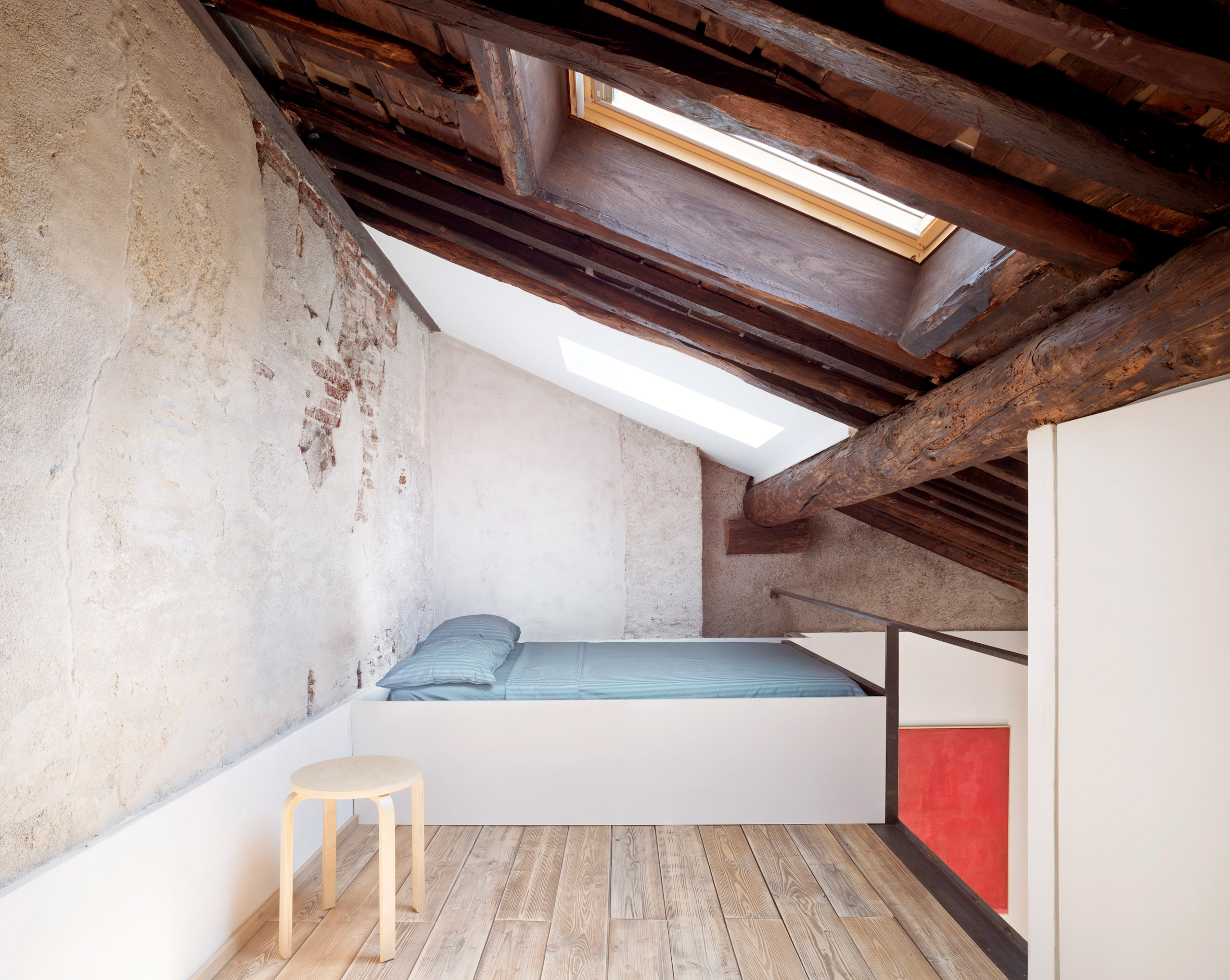The image depicts an attic sleeping area with a slanted wooden ceiling featuring a skylight that allows sunlight to stream in. Dominating the back of the room, there's a small built-in bed with blue sheets and blue pillows, nestled against a white bed frame that matches a white border running along the bottom of the room's walls. The walls are partially in disrepair, revealing red bricks beneath the damaged concrete. A wooden stool stands on the left, near a section of the exposed brick wall. The ceiling is traversed by a wooden beam adding rustic charm to the space. A metal railing extends from the end of the bed, suggesting an elevated area or loft. The wooden floor complements the warm tone of the ceiling beams. The right wall is intact and painted white, offering a clean contrast to the textured, aged left wall. The sunlight pours through the skylight, illuminating the compact, cozy space ideal for a child's sleeping area.